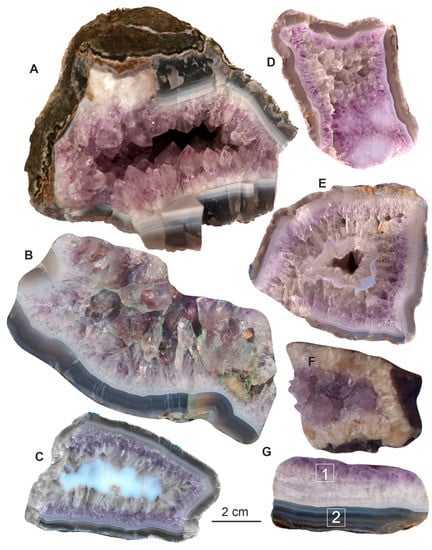The image showcases seven sliced geodes, revealing their intricate crystalline structures. The geodes are arranged in two columns—three on the left labeled A, B, C, and four on the right labeled D, E, F, G. Each geode is distinct in color, size, and shape, ranging from approximately 6 to 8 centimeters in size. The crystalline interiors predominantly feature hues of purple, with some exhibiting pinkish or bluish tones. The outer edges are dark and rugged, contrasting with the sparkly inner sections. Notably, the geode in the bottom right (G) has a unique two-tone interior, with a purple upper section and a green lower section separated by lines. A scale at the bottom center of the image indicates a length of two centimeters, providing context for the geodes' sizes. The background is stark white, emphasizing the vibrant colors and details of each rock.